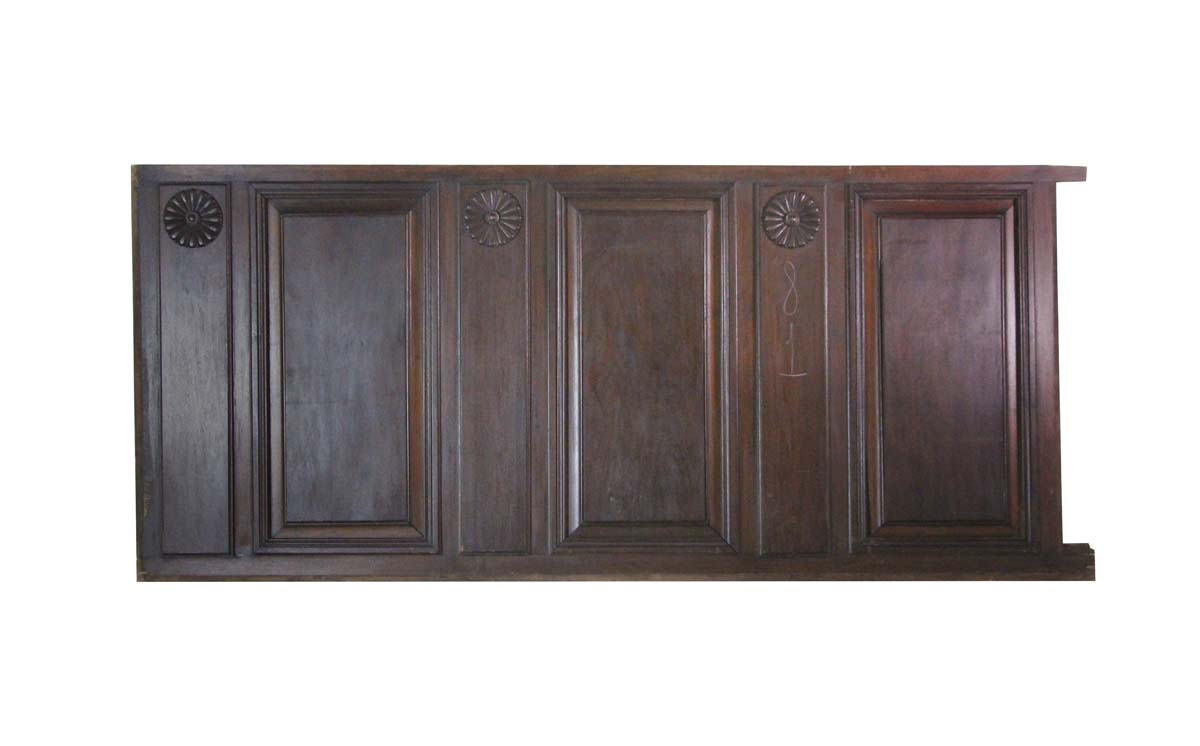The image features a close-up of a dark brown wooden piece, possibly a cabinet or wooden paneling. The wood is rich in color, exhibiting various shades of brown, and the overall design is simple yet distinctive. This wooden piece lacks handles, suggesting a minimalist style or an antique nature. Intricately etched into the front are the numbers "8" and "1." These numbers seem to be hand-carved, adding a rustic touch to the piece. The top part of the wood showcases three repeated designs, which resemble sunflower petals or floral patterns, each flanked by rectangular frames that provide a sense of depth. The combination of the etched numbers and floral motifs suggests a blend of functional labeling and decorative artistry, lending the piece an old-world charm.